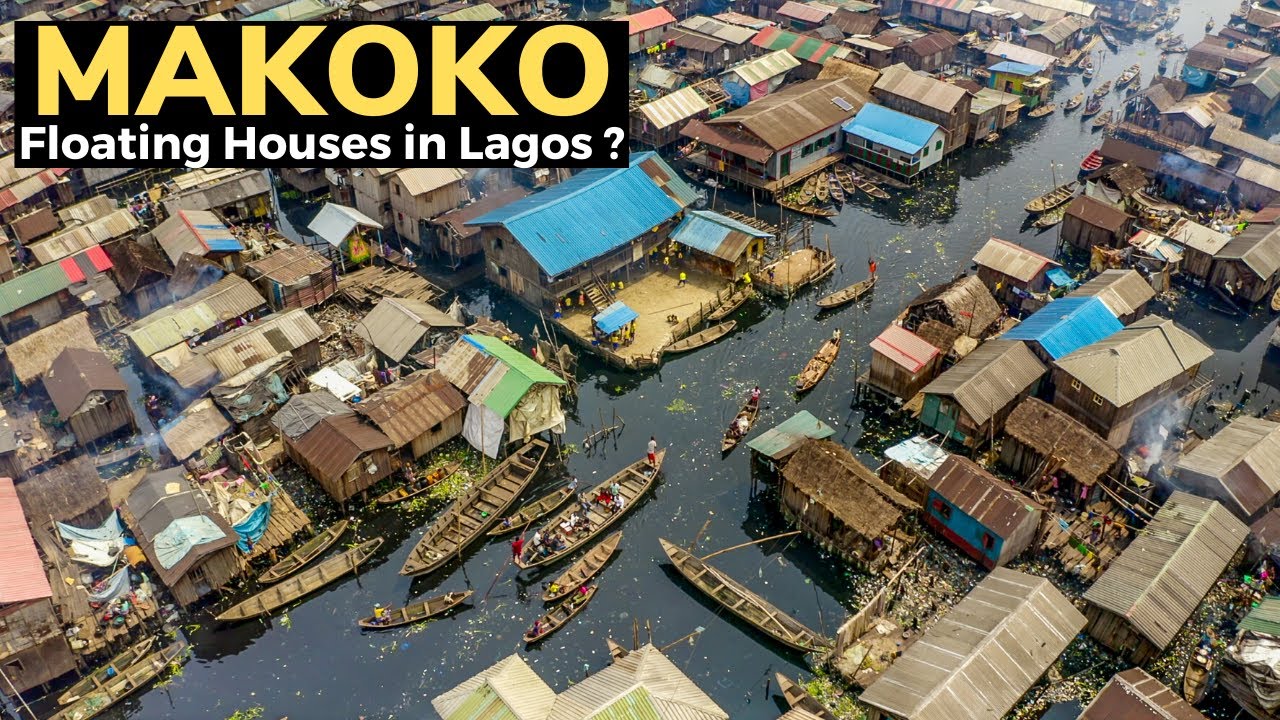In the image titled "Makoko Floating Houses in Lagos," vivid colors of blues, lime green, light pink, brown, darker brown, red, forest green, and yellow paint a visually striking scene. The photograph captures an aerial view of the floating village of Makoko, situated on a dark, almost black body of water. The village features an array of homes constructed from straw and wood, some with turquoise blue roofs and others with more traditional brown rooftops. Many of these structures appear to be in disrepair, with some roofs sinking inward, suggesting the houses have been victims of flooding or severe weather. In the top left corner of the image, a label reads "Makoko Floating Houses in Lagos." Dotted among the homes are numerous wooden canoes, in which villagers can be seen paddling. Some of these boats might belong to vendors selling goods, lending a bustling, market-like atmosphere to the scene. In summary, the image offers a poignant glimpse into the everyday life and challenges faced in this unique aquatic community.